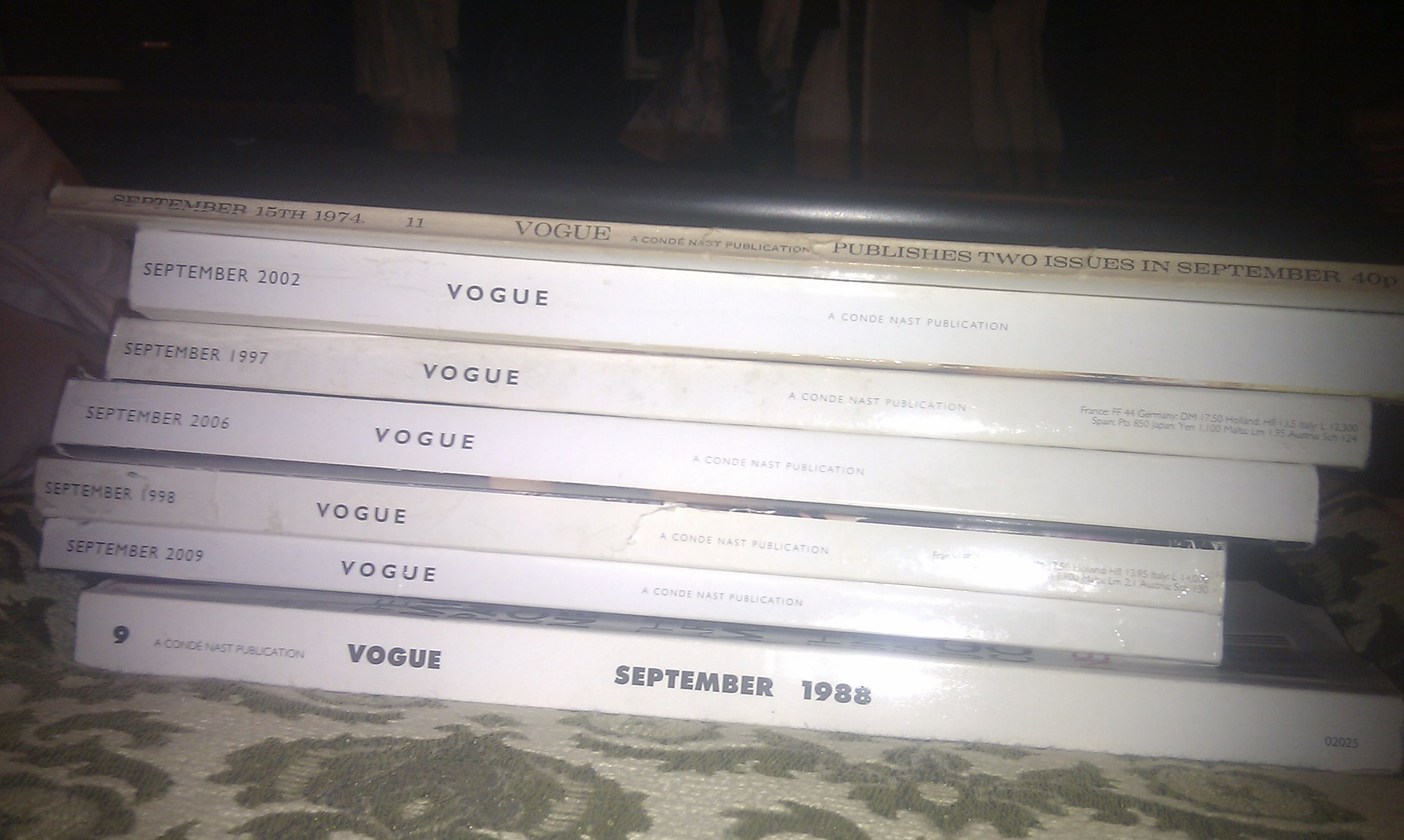The image features a vibrant green couch, identifiable by its visible backrest, against what appears to be a white wall. Resting on the couch is a collection of seven Vogue magazines, meticulously arranged in a stack with only their spines visible. The magazines vary in thickness and condition, reflecting their ages. Notably, all issues are from September, a month of apparent significance.

At the bottom of the stack is the thickest magazine, dated September 1988. Above it, in ascending order, are issues from September 2009, September 1998, September 2006, September 1997, and September 2002. Crowning the pile is the oldest issue, from September 15, 1974, which is the thinnest and most worn, indicating extensive readership. The green fabric beneath the stack, possibly with a paisley design, adds a textured background to this detailed display of vintage Vogue magazines.